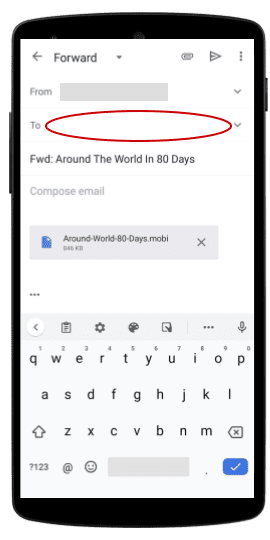In the image, there is a mock-up of an email interface displayed on a cellphone screen. The cellphone has a black exterior frame with a small button on the right-hand side near the top and a larger button on the left-hand side positioned about three-quarters up. The screen is predominantly white, featuring a gray back arrow and text reading "Forward". Icons for an attachment, compose, and a three-dot menu for additional options are also visible.

The interface showcases an empty "From" field with a drop-down menu and an empty "To" field, similarly accompanied by a drop-down menu. A red oval highlights the "To" field area. Below this, the text "Forward: Around the World in 80 Days" is visible, along with the file name "aroundtheworld80days.mobi" and a "..." indicating there is more content. 

At the bottom of the screen, a digital keyboard is displayed, resembling a typical QWERTY layout. The top row of the keyboard includes the keys Q, W, E, R, T, Y, U, I, O, P. The middle row contains A, S, D, F, G, H, J, K, L, and the bottom row features Z, X, C, V, B, N, M.